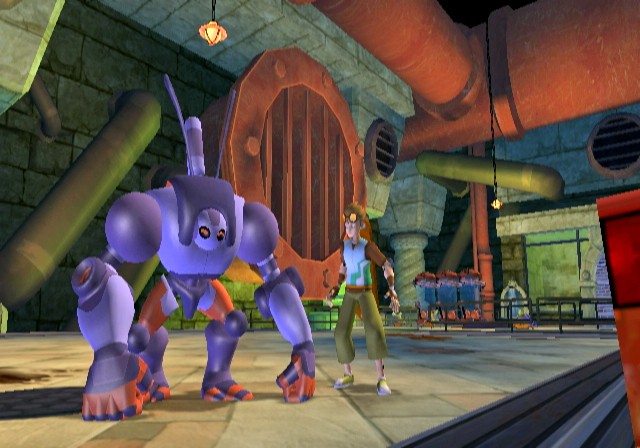A highly detailed digital image or video game screen capture depicts an underground structure, resembling a sewer or subterranean facility. Prominently featured in the upper right corner are large, cylindrical orange pipes; one extends from the right and vanishes into the background, while another perpendicular pipe emerges and exits the frame at the top. 

In the lower center-left of the image, a robotic creature stands on a stone floor. This humanoid entity, with arms, legs, and a torso, has a head embedded in its chest. Its design is sleek and mechanized, characterized by smooth shoulders and knees, with fists planted on the ground, displaying its black eyes.

To the right of this robotic figure is a character who appears to be a creator, scientist, or technician. Dressed in green pants, a white shirt with brown sleeves, and adorned with orange goggles resting on his forehead, he gazes intently at the robot. 

The backdrop features a large, vertical storm sewer grate, also orange, with five or six vertical bars. In the lower right corner, there is a bustling manufacturing area or laboratory, housing other robots that resemble the one standing in the foreground. This scene vividly captures the intricacies of a scientist's lair or a high-tech underground workshop.